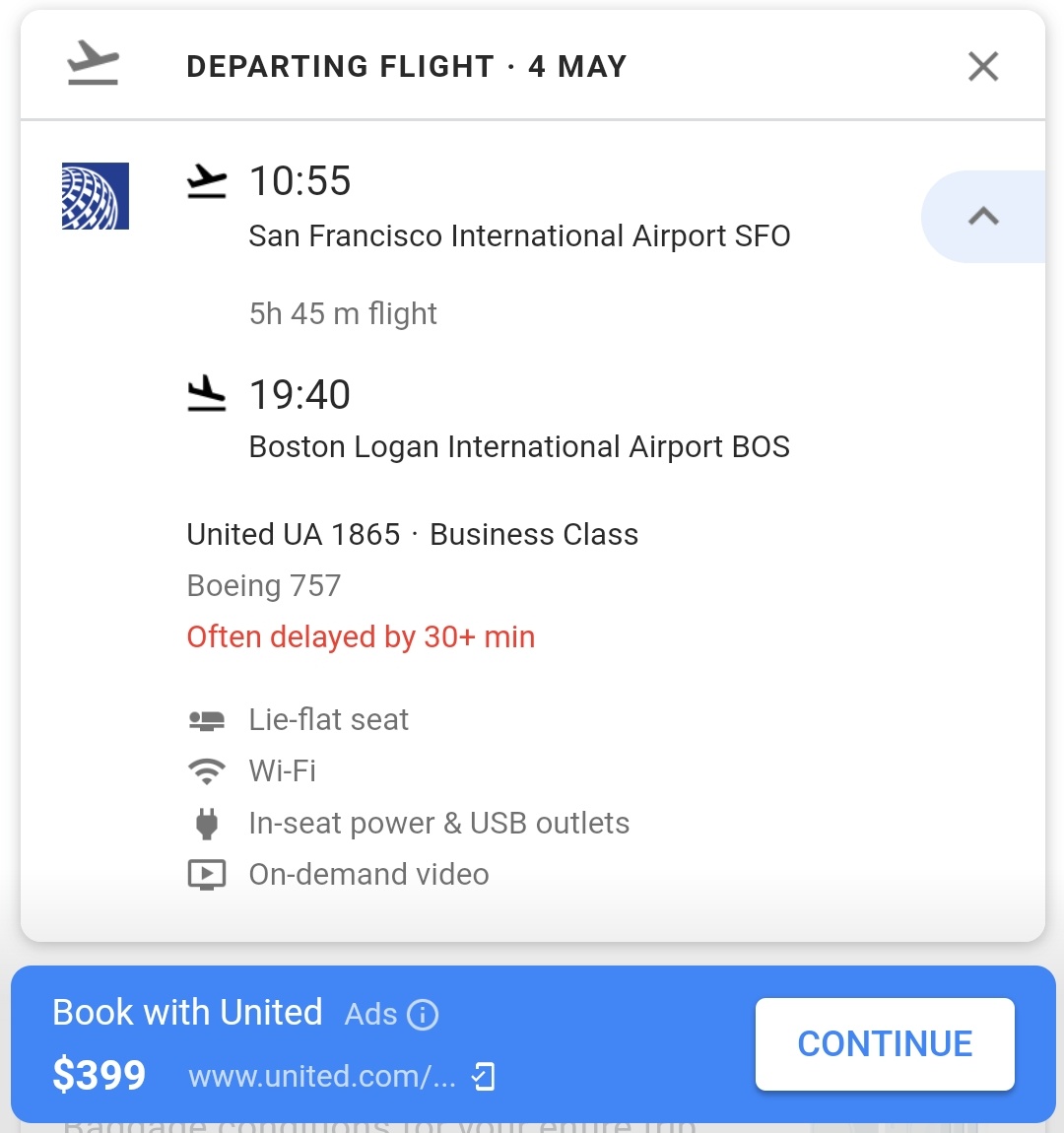The image depicts a travel itinerary with a white background. At the top, there is an airplane icon next to the text "Departing Flight for May" with an "X" symbol on the right. Below, the details are as follows: 

- Departure Time: 10:55 AM
- From: San Francisco International Airport (SFO)
- Flight Duration: 5 hours 45 minutes
- Arrival Time: 7:40 PM
- To: Boston Logan International Airport (BOS)

The next section shows the airline and flight information:

- Airline: United Airlines
- Flight Number: UA 1865
- Class: Business Class
- Aircraft: Boeing 757 (in gray text)
- Delay Information: Often delayed by 30+ minutes (in red text)

Additional amenities and features are listed in gray text:

- Lie-flat seats 
- Wi-Fi 
- In-seat power and USB outlets
- On-demand video

At the bottom, there is a blue box with the following booking information:

- Text: "Book with United"
- Price: $399
- Website: [www.united.com](http://www.united.com)
- A white "Continue" button is located on the right side.